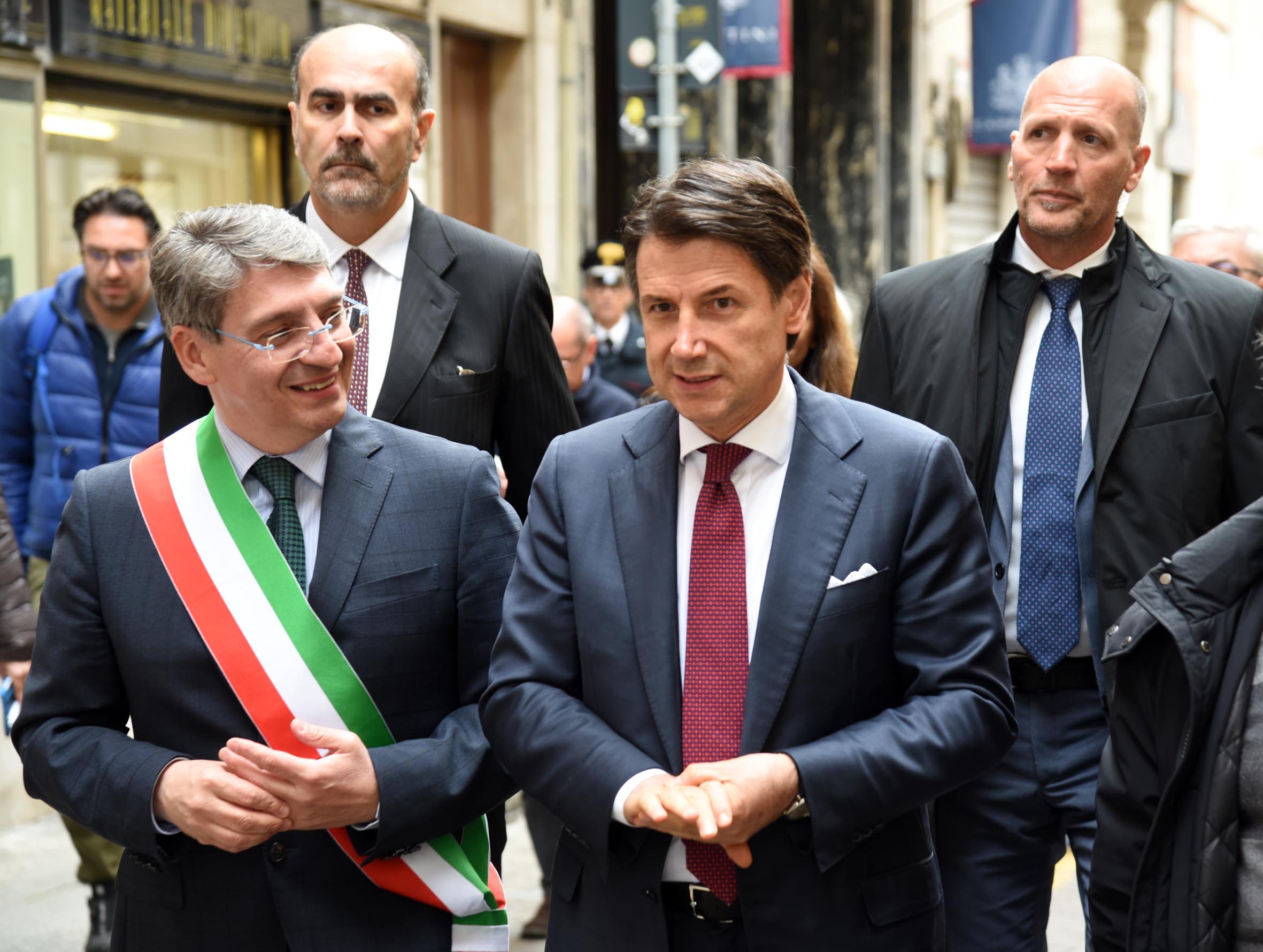In this image, we see a group of six to eight individuals, predominantly males, standing and walking towards the camera on what appears to be a stone-tiled ground in a downtown area. The setting is outdoors during the middle of the day, possibly during some kind of event. In the foreground, two prominently positioned men are wearing light blue suits; one drapes a red, white, and green banner across his chest, while the other pairs his suit with a rust-colored tie. Behind them, two large, muscular men in dark suits, who may be bodyguards, are also noticeable. Additional people can be seen in the background, though they are less distinct. The scene also features buildings in the background, though no text or wording is present in the image. The colors observed in the photo include shades of gray, black, white, dark blue, royal blue, tan, maroon, and green.